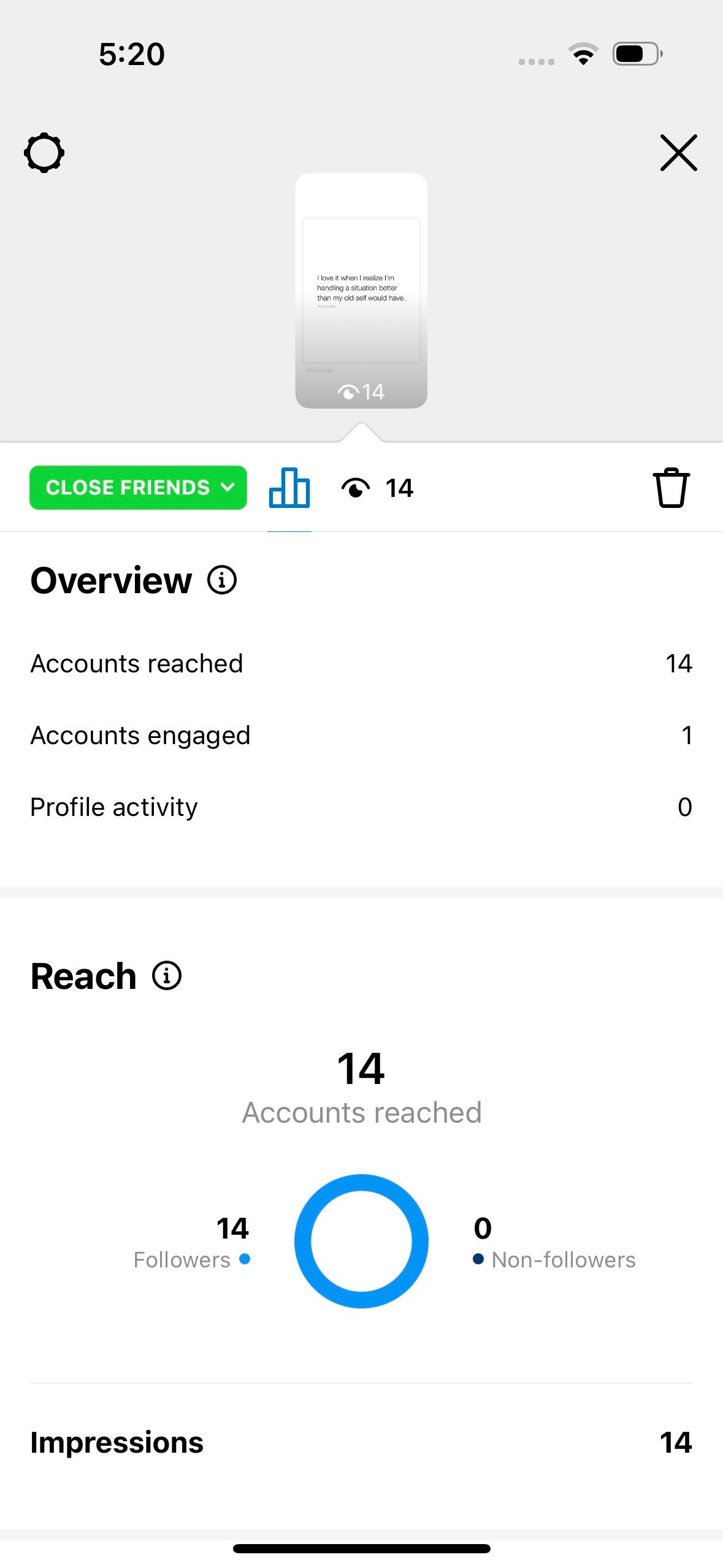**Detailed Caption:**

The image appears to be a screenshot from a social media analytics dashboard. At the top of the image is a gray rectangle displaying "5:20" on the left-hand side, with four small gray dots, a Wi-Fi symbol, and a battery indicator on the right-hand side.

On the left side of the image, below the top bar, there is an icon resembling a gear shift followed by an X. Below this, there's a large rectangle that starts white at the top and gradients to gray at the bottom. In the center of this rectangle, there is textual content, along with a white symbol showing the number "14." 

Beneath this, there is a green rectangle labeled "Close Friends," followed by an unidentifiable symbol. Adjacent to this section are three vertically aligned blue-outlined rectangles; the middle one is notably the tallest.

Further down, there's a black curved line paired with a partial circle beneath it, displaying the number "14." Right next to it, there is an icon resembling a trash can. Below this series, a thin gray line spans the width of the image.

The title "Overview" is prominently displayed, followed by a gray-outlined circle featuring an "I." The text "Accounts Reached" appears along with the number "14." Underneath are the metrics "Accounts Engaged" with a value of "1" and "Profile Activity" with a value of "0."

A thin gray rectangle separates these sections from the subsequent text, which reads "Reach," along with a circle either outlined in black or gray containing an "I." This is followed by "14 Accounts Reached."

On the left-hand side, the number "14" is shown followed by "Followers" with a blue dot adjacent. There is also a blue-outlined circle next to the number "0." Beside this, a dark blue circle is labeled "Non-Followers."

A light gray line runs across the image above the "Impressions" section, which states the number "14." Another light gray line is placed underneath, followed by a final black line at the bottom of the image.